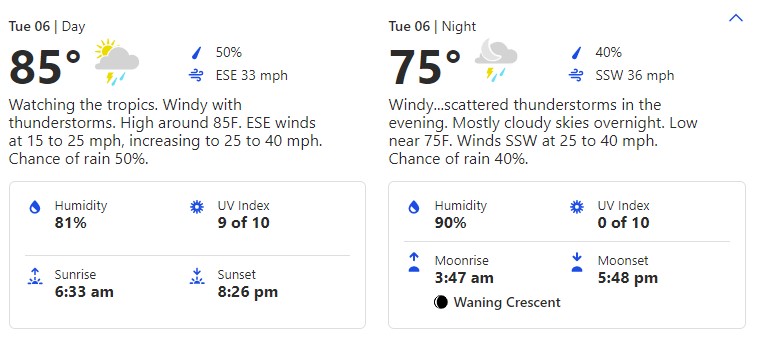This image presents a weather report for Tuesday, June 6th, divided into two sections: day and night.

On the left side, the daytime weather is highlighted. The report indicates:
- **Temperature:** 85°F
- **Precipitation Probability:** 50%
- **Wind:** East-southeast at 33 mph 
- **Additional details:** 
  - **Humidity:** 81%
  - **UV Index:** 9 out of 10
  - **Sunrise:** 6:33 AM
  - **Sunset:** 8:26 PM

An accompanying illustration depicts a cloud with raindrops and the sun partially obscured behind it, symbolizing potential rain showers.

On the right side, the nighttime weather details are provided:
- **Temperature:** 75°F
- **Precipitation Probability:** 40%
- **Wind:** South-southwest at 36 mph 
- **Additional details:** 
  - **Humidity:** 90%
  - **UV Index:** 0 out of 10
  - **Moonrise:** 3:47 AM
  - **Moonset:** 5:48 PM

This section includes an image of a cloud with raindrops, indicating a chance of rain during the night.